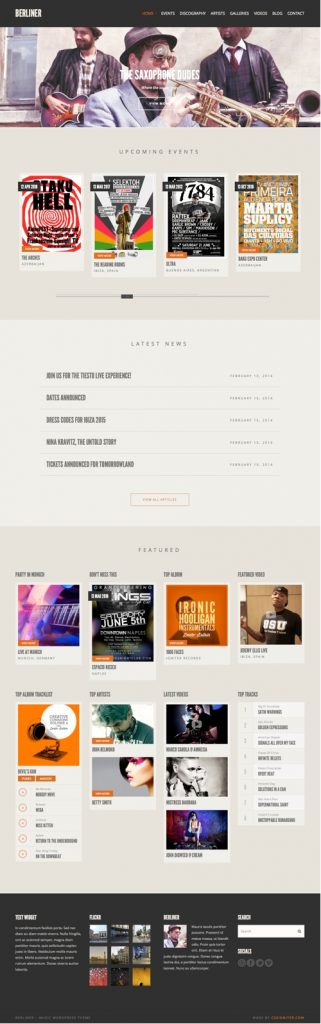The image appears to be a zoomed-out screen capture of a vibrant and diverse website layout. The top of the page features a thin black line with a white logo positioned prominently, followed by a series of white submenus. 

Below this header, there's a central image featuring three men. Two of them are dressed in suits, while the third is more casually attired. The middle of the image contains the text "The Saxophone Keys" in white. The man at the forefront wears a brown hat, sunglasses, and a gray sport jacket. He is holding a gold saxophone. Behind him is another man in a black jacket, sporting a burgundy tie and a black vest. Over the shoulder of the man with the hat, a third individual is visible, dressed casually in a plaid shirt and black jacket, and appears to be holding a guitar.

Further down the page, various images are displayed in a series:
- A black, orange, and white image with the text "Taco Hell."
- A multicolored image (black, white, pink, gold, and green) featuring someone's handwriting.
- A black and white image displaying the numbers "7784."
- A yellow, green, and orange image with the text "Marta Suplicy."
- A tan box outlined in black, followed by a section titled "Latest News" with a list of items in black text.

After the news section, additional colorful images are arranged:
- A purple and pink image with black font.
- A black and white image with the date "June 5th."
- An orange image with white text.
- A man in a black shirt featuring white icons.
- An orange image with a white speech bubble and black text.
- A teal image depicting a woman with futuristic pink makeup.
- Black and white, black and blue, and purple images.

Towards the bottom of the page, another menu area with black font is visible, ending in a black section with white text that contains a gallery of images, including a photo of a person. A search box is positioned at the very bottom of the page, completing the website layout.

This detailed description captures the essence and intricacies of the web page, providing a vivid mental image of its content and structure.